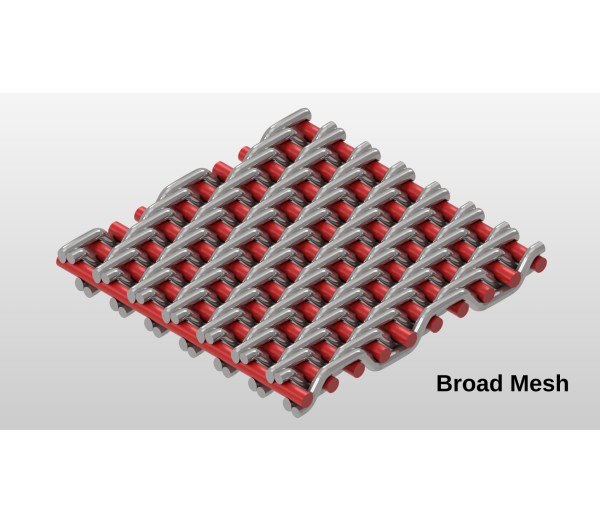The image is a detailed digital screenshot of a 3D rendered mesh material set against a grayish gradient background. The centerpiece of the image features a square-shaped metallic mesh composed of crisscrossing wires and red cylindrical rods. The gray wires follow a pattern beginning from the bottom left, weaving over and under the red rods as they span diagonally from the top left to the bottom right corner. This pattern repeats consistently across the mesh to create a broad, net-like structure. The red rods and gray wires together form a complex mesh design that closely resembles a chain-link fence with additional reinforcement bars. In the bottom right corner, the words "Broad Mesh" are prominently displayed in capitalized black font, providing a clear label for the object depicted. The overall style of the image indicates it serves as a demonstration diagram, likely modeled in 3D software.